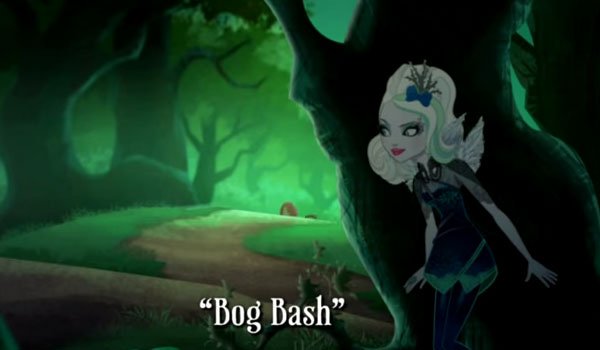The image is a still from an animated cartoon, capturing a dark, muted forest scene dominated by shades of green. In the center, white text in parentheses reads "bog bash." The setting features thick trees, their trunks dark and ominous, some glowing green on the sides. A winding dirt path meanders through the scene, with hints of figures - possibly a person and a small figure or dog - barely visible along the trail. 

On the right side of the image, partially hidden behind a dark tree, stands a female character with wavy, thick blonde hair, adorned with a purplish-blue bow and bits of green foliage. She has pale skin, dark eye makeup, and striking red lips. Dressed in a black outfit with green trim and a zigzag bottom, she appears to be watching intently, possibly on the lookout for someone. Her pose and expression contribute to the forest's eerie, mysterious atmosphere.